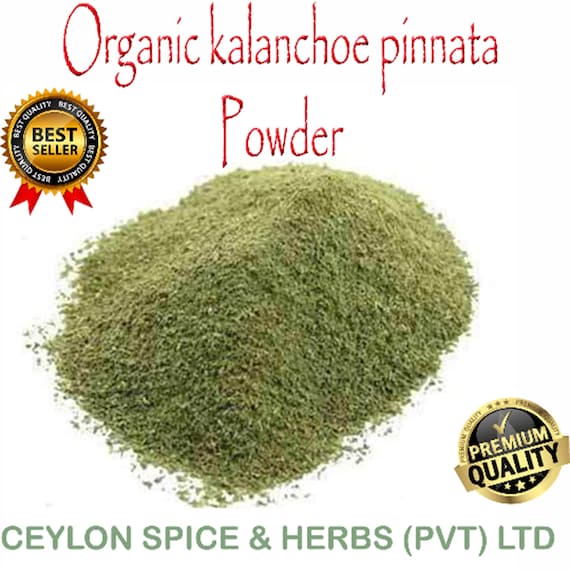The image is of a product label for Organic Kalanchoe Pinata Powder, set against a white background. The main text at the top of the label is written in red. In the center of the label, there is a heap of greenish-brown finely powdered herb. To the left of the powder, there is a gold ribbon with red detailing that reads "Best Seller." On the bottom right, there is another round seal: it features a gold-edged outer circle and a black inner circle. This seal says "Premium Quality" in gold lettering, with three stars underneath the word "Quality" and a check mark. At the bottom of the image, there is a line of text in parentheses that reads "Ceylon Spice and Herbs PVT LTD."